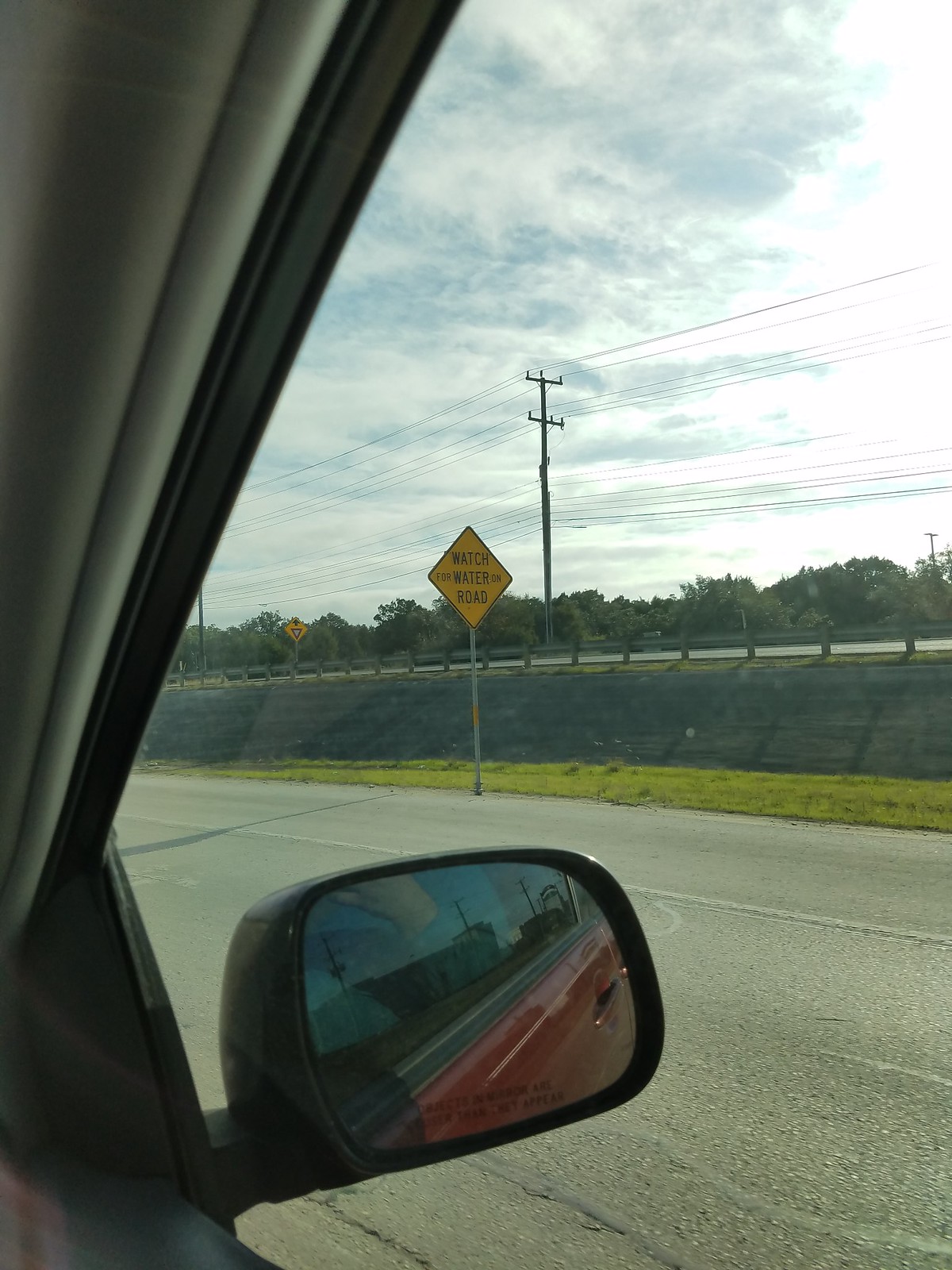A vivid outdoor scene captured from the passenger side of a red car traveling in the left lane of a highway. The photograph includes the car’s window edge, with the side mirror clearly reflecting the driver's hand and the car's vibrant red color. Positioned along the roadside is a partially visible yellow sign indicating, "Watch [Something] Road." The landscape features a grassy area leading up to an embankment, topped with another roadway, separated by a sturdy guardrail. In the background, a telephone pole rises against a sky filled with a tapestry of clouds. This detailed image underscores the dynamic interplay between human presence, automotive travel, and the surrounding environment.